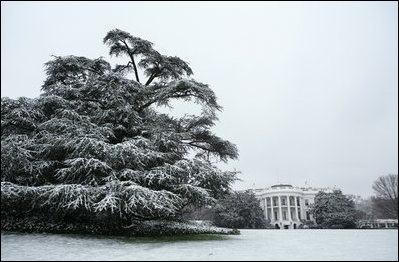This is a black-and-white photograph that prominently features a large, bushy tree in the left foreground, likely a pine tree, which has white elements due to snow particles. The tree appears dark, almost black, possibly due to post-processing effects. To the right side of the image, the White House is partially visible, characterized by its white facade and iconic round columns. The building is framed by two additional trees, one bare and another densely foliaged. A flat, expansive, snow-covered lawn extends towards the White House, emphasizing the distance from which the photo was taken. Above, the sky appears clear and contributes a light backdrop to the scene. A thin black border frames the entire image, enhancing its classical black-and-white aesthetic.